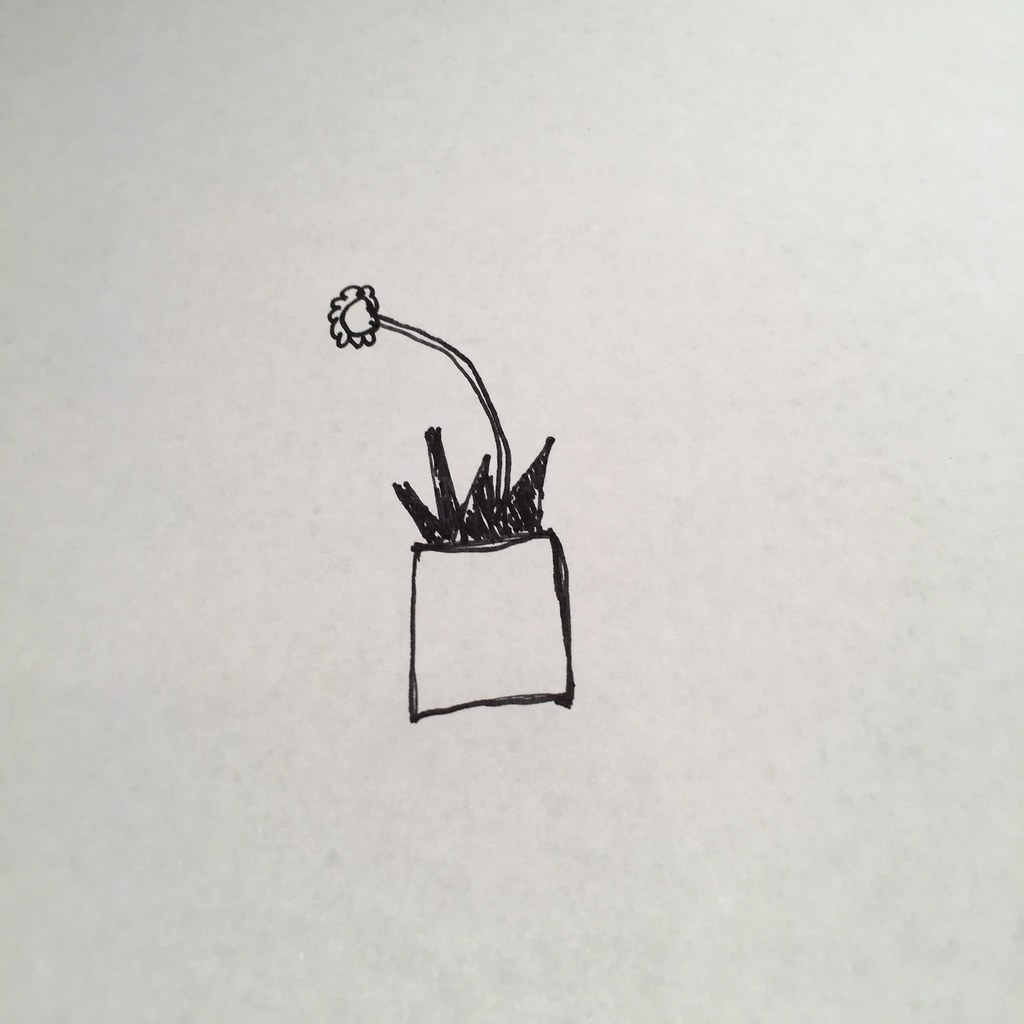The image is a black pen drawing on white paper, featuring a simple and whimsical illustration of a potted flower. The flower emanates from a tall, curving stem that bends gracefully towards the left. At the top of this stem is a bloom with a large, circular center surrounded by numerous small petals, resembling a poppy. The flower pot is a small, roughly outlined square with slightly curved edges, positioned prominently in the middle of the paper. Inside the pot are several leaves, some triangular and others rectangular, all filled in with dark ink. Additionally, the pot has four tall, pointed structures on top, reminiscent of a crown, with the second point from the right being the tallest, indicating a simplistic yet imaginative design. Despite the lack of shading on the flower and its stem, certain elements like the crown are shaded, giving it a dynamic, handcrafted feel. The overall drawing carries a childlike spontaneity, making it appear both natural and intentional in its simplicity.